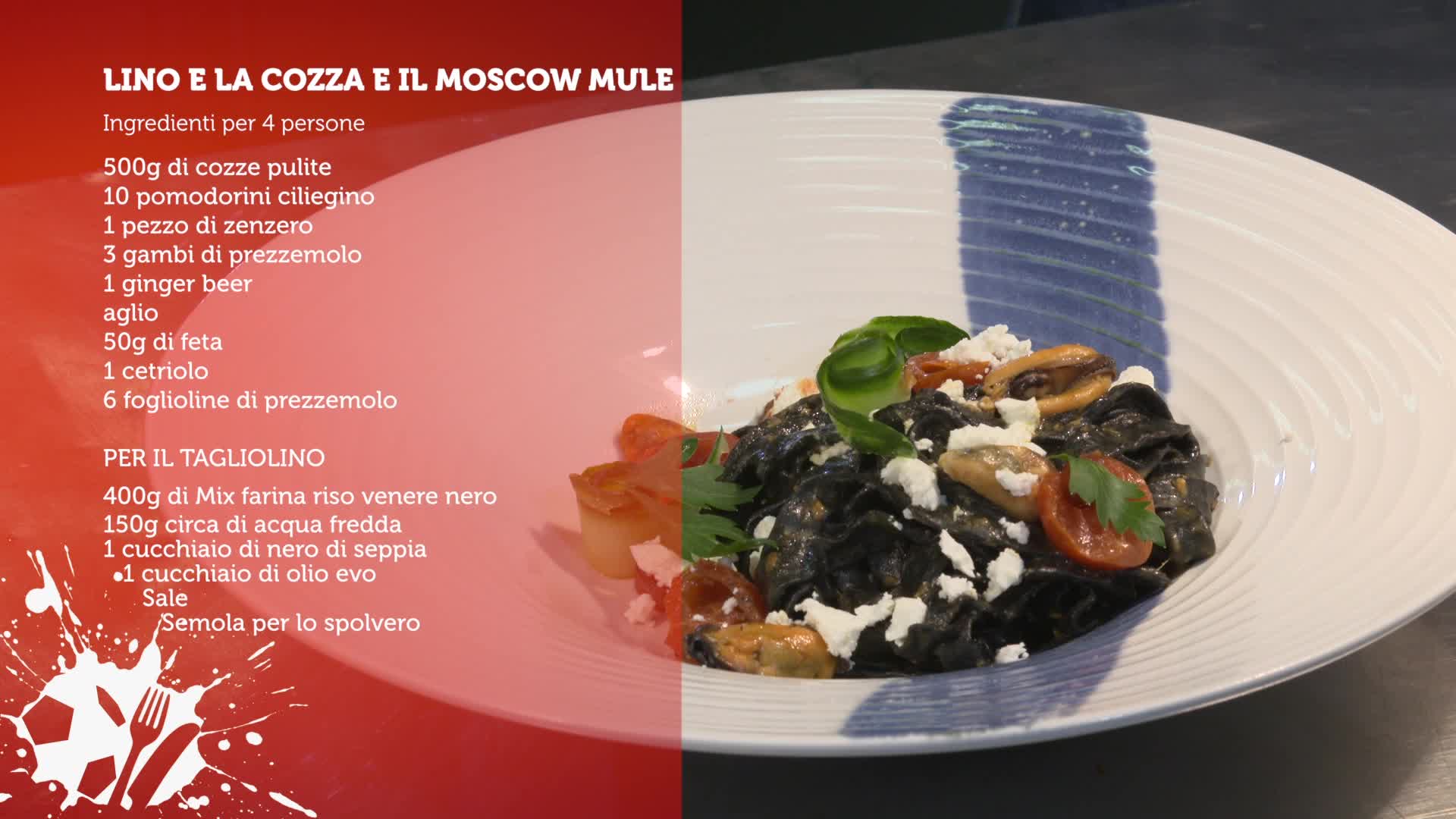The image features a visually appealing infographic that appears to be targeted for social media or a food blog, possibly Instagram. At the center of the image, there is a concave, white salad plate with a distinctive blue stripe painted across it. The plate holds a vibrant salad consisting of assorted mushrooms, sliced tomatoes, green vegetables—likely cucumber slices—purple and green leafy greens, and sprinkled crumbled cheese. Interestingly, a few nuts are also visible, adding texture and variety to the dish.

To the left of the plate, there is an overlaid, translucent red infographic written in Italian. Despite being see-through, allowing the plate to remain visible, this section details a recipe. The text atop says "Lino e La Cosa il Moscow Mule," followed by a list of ingredients and preparation instructions, presumably for a Moscow Mule cocktail. Although the primary visual focus is the salad, the juxtaposition with the Moscow Mule recipe creates an intriguing and slightly puzzling combination of food and beverage presentation.